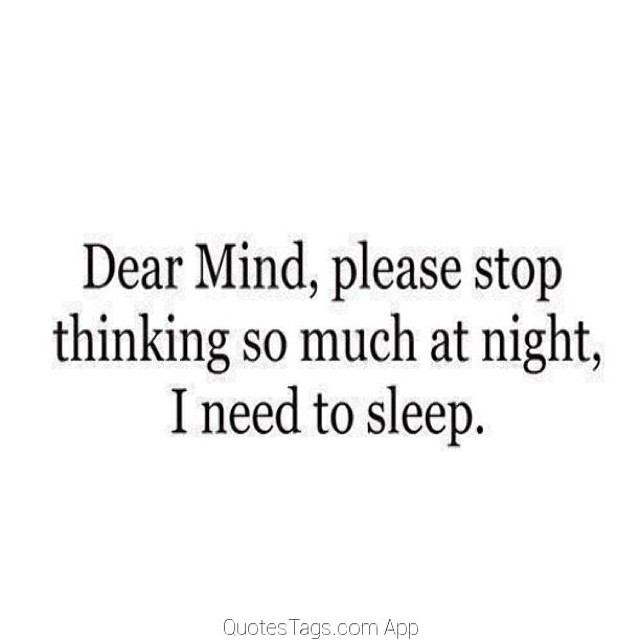The image features a completely white background with minimal black text in the center, spanning three lines. The message reads, "Dear Mind, please stop thinking so much at night, I need to sleep." The text is centered both horizontally and vertically within the image, with ample padding at the top and bottom. Capital letters are used for "Dear" and "Mind," and a comma is included after "night." A light gray web address, "quotes tags.com app," is placed at the bottom of the image. There are faint light gray highlights around some characters within the central quote text. The image exudes a sense of simplicity and focuses on conveying the relatable plea of a person addressing their overactive mind at night.